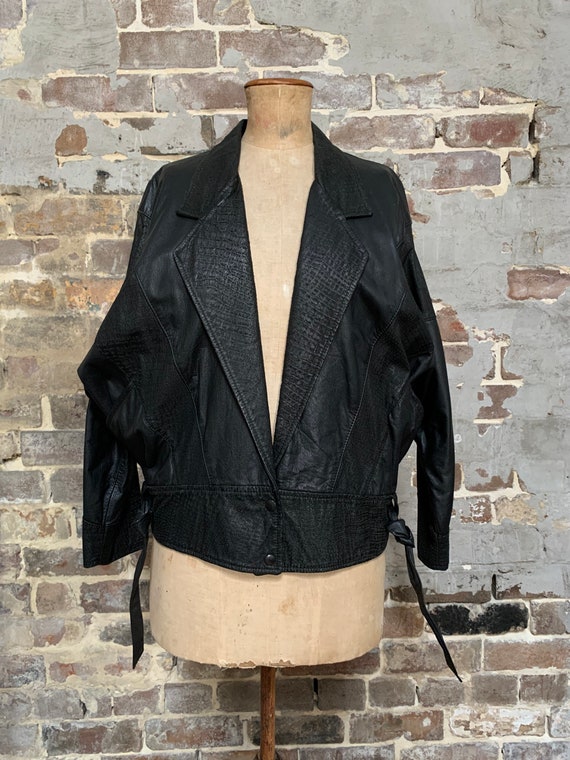The photograph showcases a black leather jacket displayed on a headless mannequin. The mannequin, supported by a wooden pedestal extending from a thin brown pole, has a neck and a torso that ends well past the waist, with no legs. The jacket features an open V-neck design, with a normal collar, long sleeves, and a couple of buttons near the bottom. Straps hang down from both sides of the lower part of the jacket, suggesting a possible feminine style. The backdrop is a rustic brick wall partially covered with worn and removed stucco, revealing the mortar between the bricks. The lighting is sufficient to highlight these details, with a focus on the jacket. The photo appears to be taken indoors, with the photographer standing and capturing a straight-on view of the mannequin. The colors in the image include shades of brick red, tan, beige, gray, and black, creating a visually balanced composition.